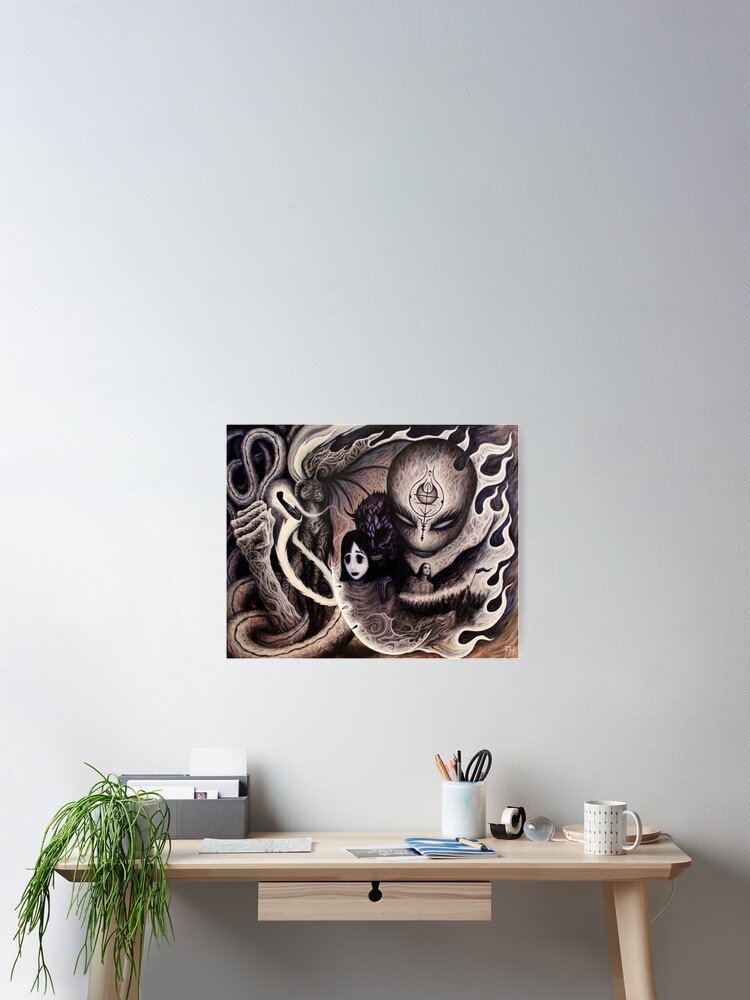The photograph showcases a contemporary, minimalist desk setup set against a large, blank white wall. The focal point on the wall is a distinctive piece of artwork depicting a supernatural scene with a face encircled by flames, arrows, and serpentine shapes, rendered in black, brown, and white, evoking a slightly eerie ambiance. The desk, made of smooth light wood, features a simple design with one small drawer and four legs, maintaining an organized and clutter-free appearance. On the desk's surface, at the front left corner, sits a small green plant adding a touch of nature. Towards the back, there's a gray filing organizer, suited for mail or other documents. Various office supplies are meticulously arranged, including a white cup holding pencils and scissors, a black tape dispenser with clear tape, and a white coffee mug with some drawing on it. A sleek, white articulated desk lamp is perched on the right side, completing the modern aesthetic of this workspace.